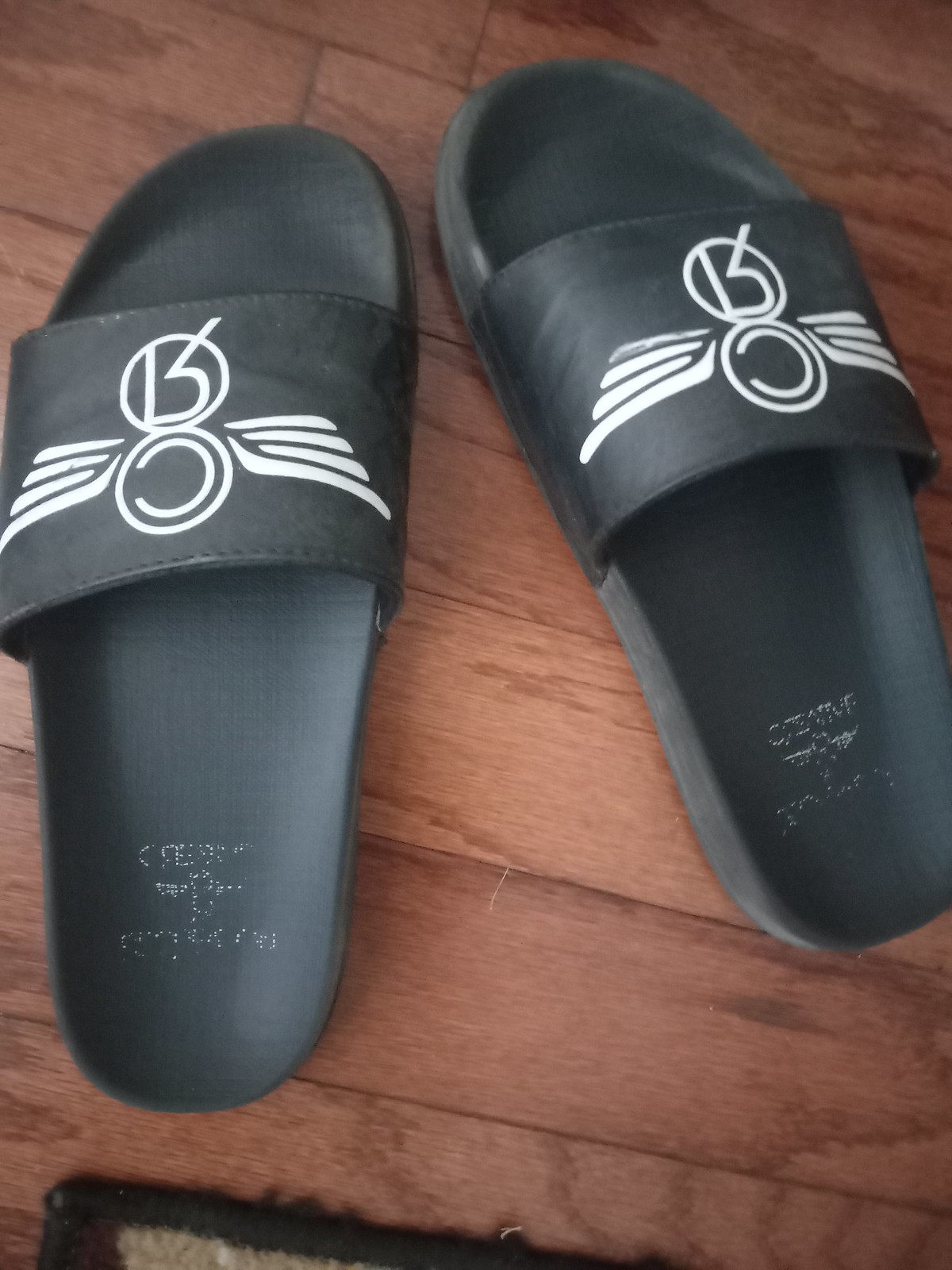This detailed photograph captures a pair of black flip-flop slippers, prominently displayed on a medium-toned wooden floor. The floor features darker brown lines and black creases where the wood pieces meet. At the very bottom edge of the photo, there's the border of a carpet, which is primarily black, with beige and maroon fibers catching the light.

The flip-flops are constructed from black rubber, potentially with a leather-like appearance, featuring a simplistic design with minimal coverage over the feet. Notably, the top part of each slipper has a distinct branding detail: two white circles stacked vertically. The upper circle has an inverted 'R,' and the lower circle features a 'C' facing left. Extending from either side of these circles are stylized wings, reminiscent of bird or angel wings. This white decal is slightly worn, indicating regular use.

At the heel of each flip-flop, there's a faded white logo, which suggests it once read "Creative", though it’s mostly rubbed off now. The overall condition of the flip-flops shows signs of wear, such as light dust and scuffs, further emphasizing their frequent use.